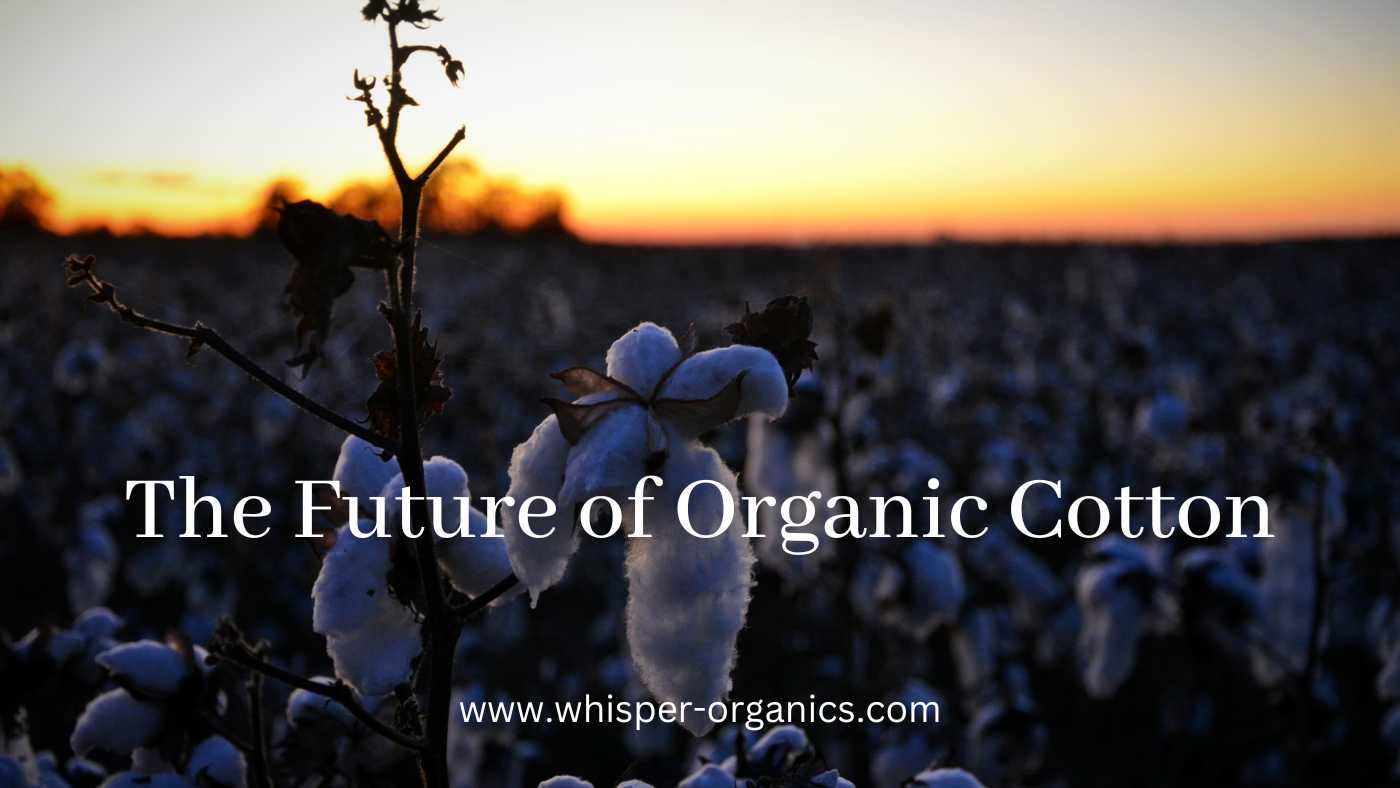The image is a rectangular banner for a blog or web page, set in a landscape layout where the top and bottom edges are longer than the sides. The background features a large field of cotton plants ready for harvest, with numerous long brown stems sprouting from the ground and supporting sagging white cotton bolls. The scene is bathed in the warm hues of a sunset, with the top 20% of the image transitioning from white to yellow and then a deep orange, while the bottom part grows darker, almost black. On the left side, a twig ascends and partially obscures the bright sky. Overlaying the image, in the center, are white text captions: "The Future of Organic Cotton" with each initial capitalized, and at the very bottom, the website "www.whisper-organics.com" in lowercase letters. This banner serves as an advertisement for organic cotton, emphasizing the serene and natural beauty of the field during sunset.